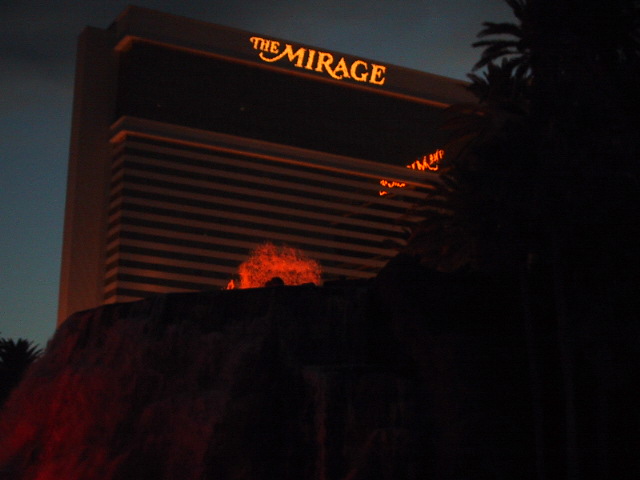This photograph of The Mirage hotel and casino in Las Vegas captures a nighttime scene with limited visibility. The focal point is the illuminated sign at the top of the hotel, displaying "The Mirage" in a distinctive font, lit up in yellow against the darkness. Below the sign, the hotel extends down into the shadows, with its alternating black and white floors faintly visible. The sky around the building is a dark, gloomy gray with a hint of blue, suggesting that it might be late evening or early morning. The right side of the image shows the silhouettes of tall palm trees, adding to the tropical ambiance. The bottom half of the photograph is dominated by a large, dark structure obscuring part of the scene, potentially a fountain with water lit up in red, but the details are obscured by the night. The overall composition highlights the eerie yet captivating allure of The Mirage against a dusky Vegas skyline.